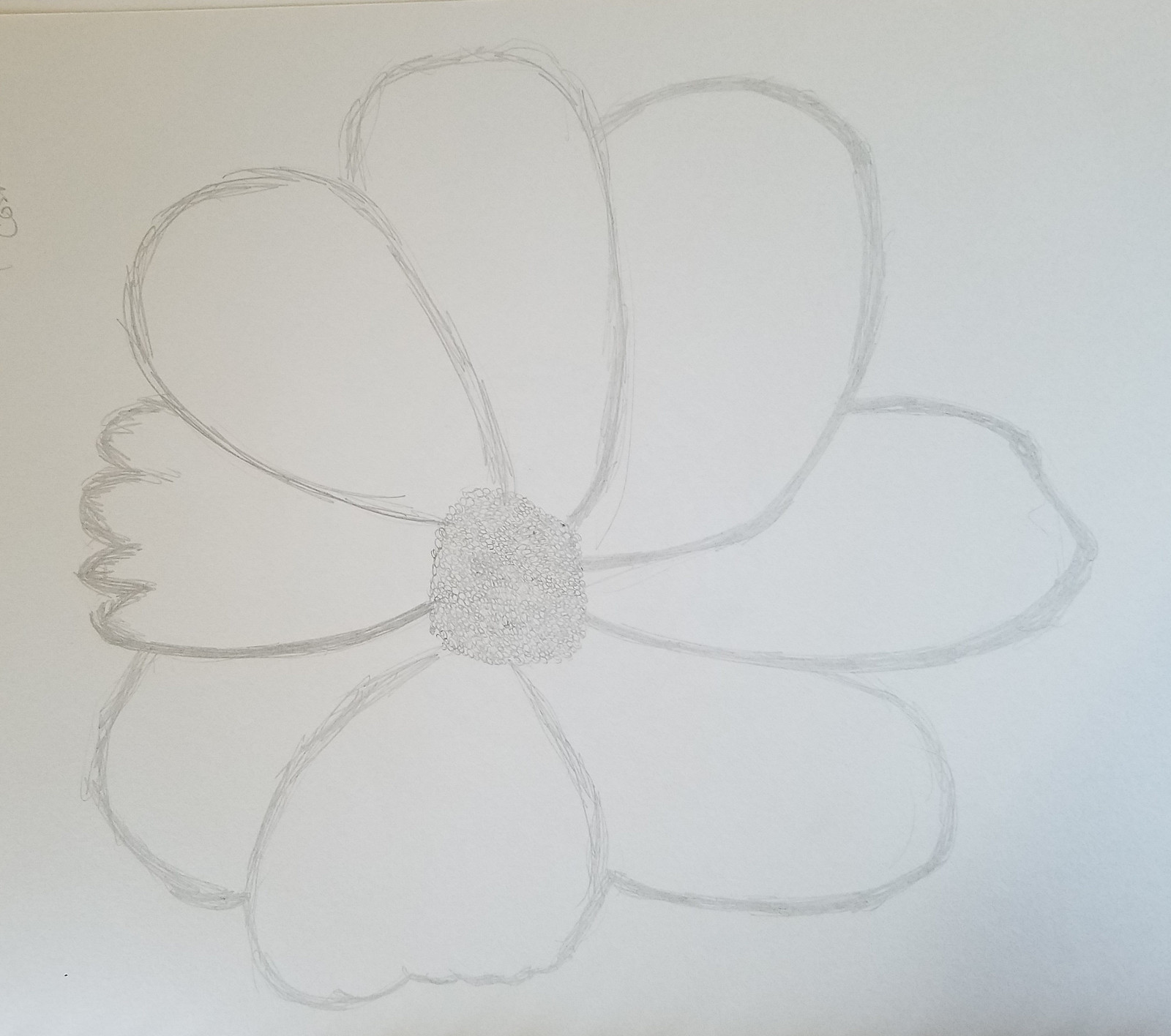This is a detailed description of a minimalist pencil sketch of a daisy. The sketch captures the essence of the daisy with remarkable simplicity and creative design choices. The majority of the petals are rounded and oval, true to the flower's natural form, but there are intriguing deviations that add character to the piece. One petal stands out with its inverted heart shape, while another features four distinct lobes at its tip, diverging from the usual petal shape. The center of the daisy is intricately detailed with a multitude of small circles, emphasizing the detailed work of the artist. The sketch, likely rendered with a sharp graphite pencil, is set against a light gray background, enhancing its minimalist appeal and allowing the unique features of the daisy to shine.